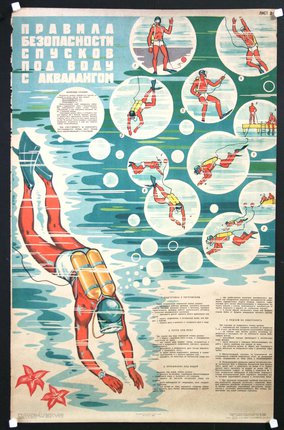This is a vintage 1970s-style Russian poster, likely an advertisement or safety diagram about scuba diving, rendered in a distinct retro design. The poster is bordered in black and features imagery central to illustrating underwater safety. Dominating the left lower two-thirds is an animated figure of a scuba diver swimming away from the viewer, with two yellow cylindrical oxygen tanks on his back, a helmet, and flippers, all accented by a red bodysuit. Bubbles rise from his equipment, each containing circular images depicting various underwater scenarios that may be encountered during a dive. A couple of starfish and two red flowers can be seen in the bottom left corner, adding to the underwater theme. The top left bears unreadable white text in what appears to be Cyrillic script, while a similar typed section in black is located in the bottom right quadrant, possibly offering detailed safety instructions. Overall, this weathered and stylistically nostalgic poster vividly captures an era-specific approach to scuba diving safety education.